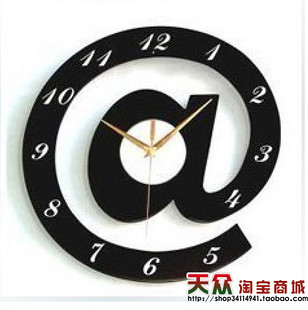This image features a distinctive black clock designed in the shape of the "@" symbol commonly used in email addresses and social media tagging. The clock face integrates white, elegantly styled numbers that follow the circular outline of the "@" symbol, but the circle doesn’t completely connect, breaking between the numbers 4 and 5. The clock’s hands—one for seconds, one for minutes, and one for hours—are placed centrally within the circular part of the "@" symbol's "A" and are crafted in gold. The current time displayed is approximately seven minutes past ten. Additionally, there are some Chinese characters written in red and black located in the bottom left corner of the image, potentially indicating the manufacturer's name or other relevant information. The clock is set against a plain white background.